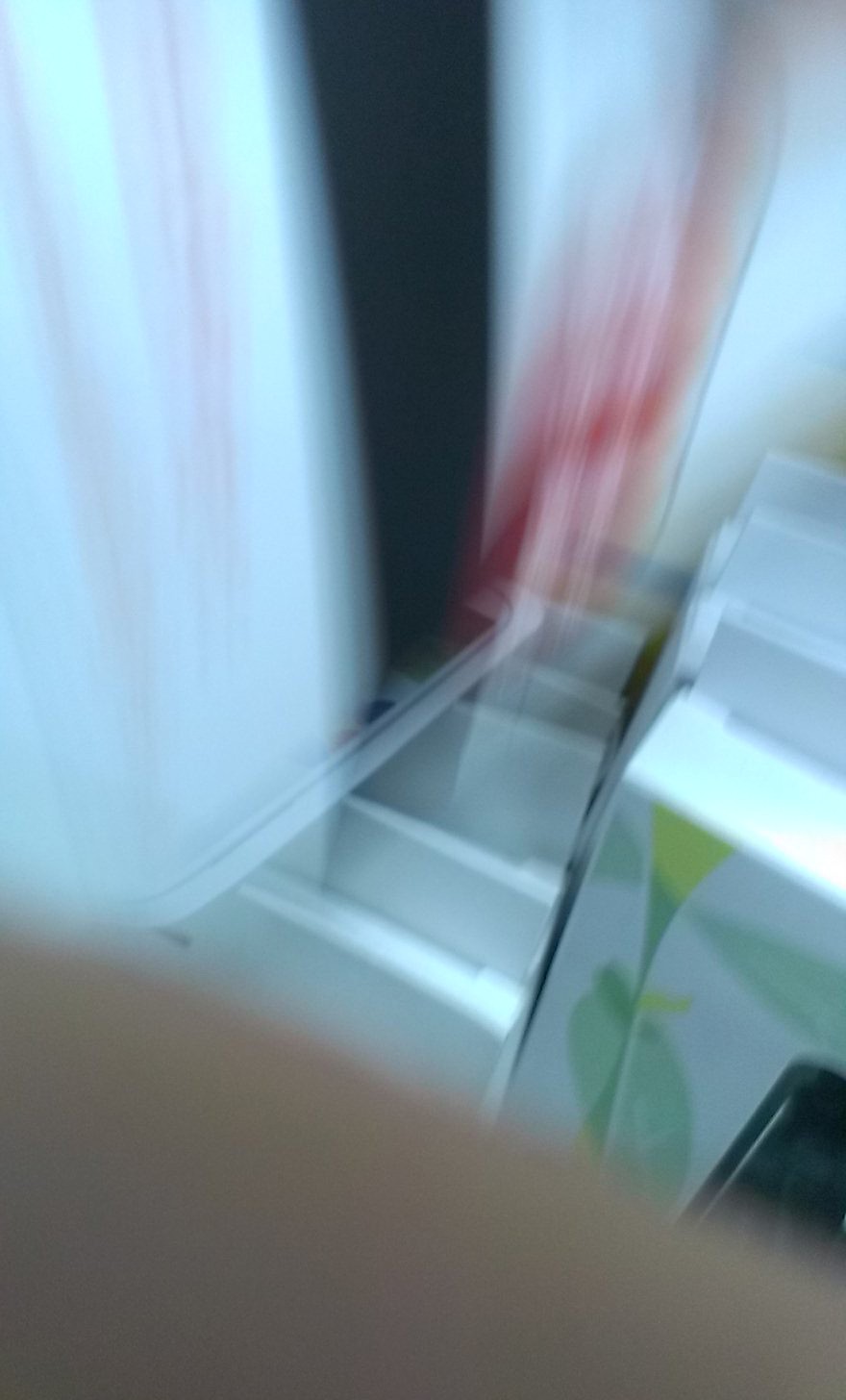In this blurry image, the right side prominently features a countertop illuminated by soft lighting. Below the countertop, a pattern of green leaves against a white backdrop is visible, adding a touch of nature-inspired decor. At the bottom, there seems to be an appliance, possibly a washing machine or dryer, indicated by the presence of a circular, hole-like feature. On the left, a black curtain or fabric is partially obscured by motion blur. In the center, a person wearing red can be seen moving across the frame. At the front, there is a indistinct white or gray object, further contributing to the overall blur and haziness of the image.